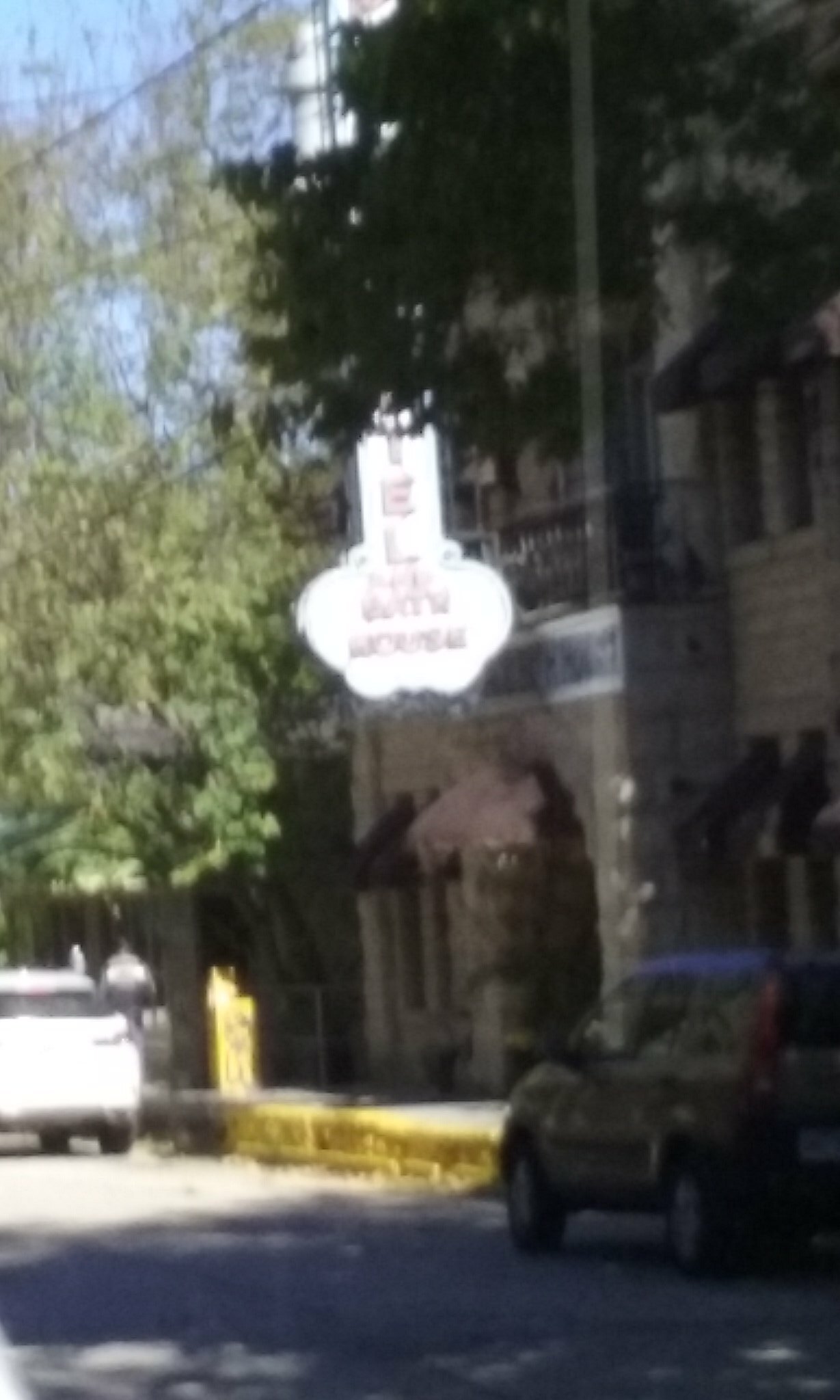The photograph is a color image in portrait orientation, taken outdoors. Despite a slight blur, several details are discernible. The background reveals a clear blue sky and distant trees casting shadows on a nearby roadway. Prominently featured is a beige brick building, likely a hotel or motel, as suggested by the red awnings out front and a sign with partially visible letters "E" and "L". A tan SUV is parked near the building. The foreground showcases a curved sidewalk leading to the building's entrance, marked with yellow caution or no-parking zones.